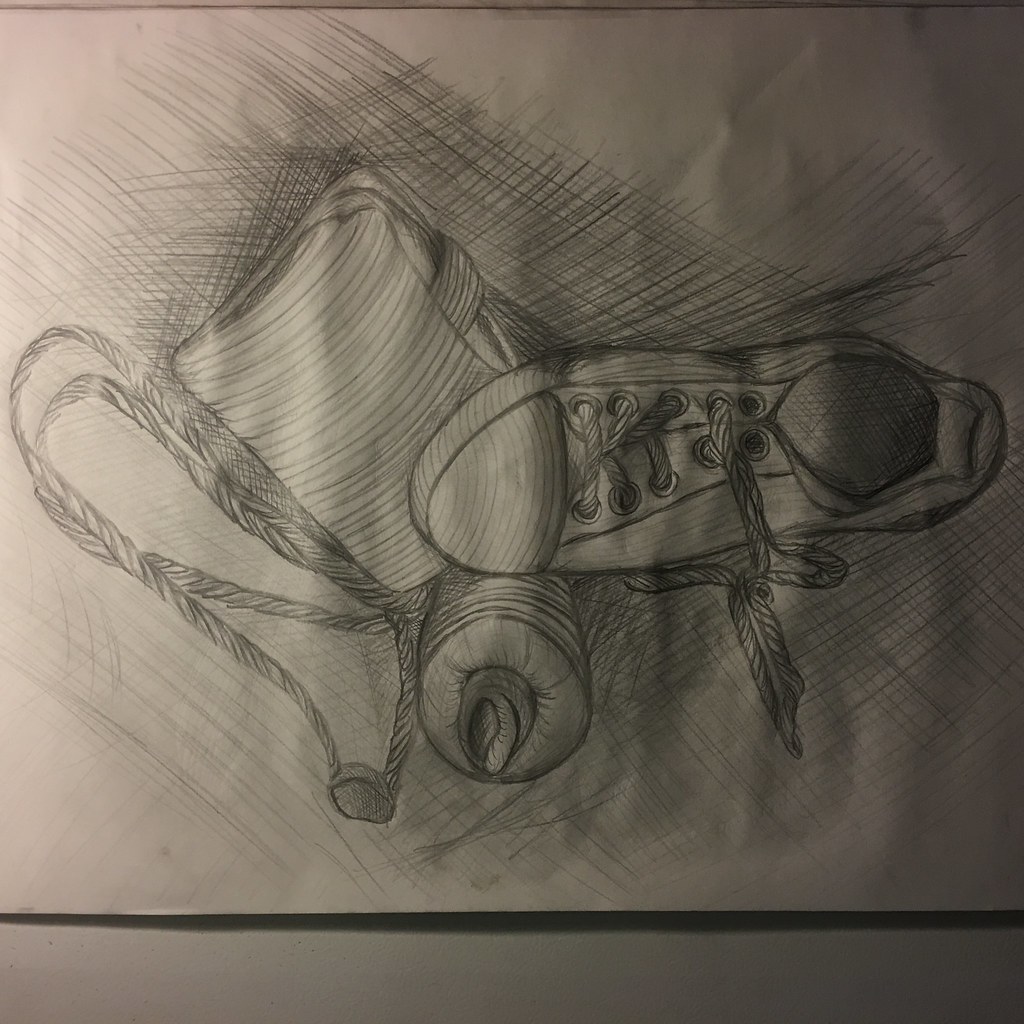The image displays a detailed pencil sketch on white paper, emphasizing a central composition of workout items. Dominating the right side is a light gray sneaker, with intricately drawn thick shoelaces criss-crossing through the bottom four eyelets, while the top two eyelets remain untied, leaving the laces loose. The shoe features a distinct striped pattern, with darker shading inside the opening and lighter tones on the exterior. Adjacent to the sneaker, there is a water bottle with a spout, supplemented by a folded, bundled towel. On the left side of the composition lies a braided rope, adding to the scene's dynamic texture. The background encompasses meticulous scratch work and shadowing, providing depth and context, as if suggesting the aftermath of an active session.